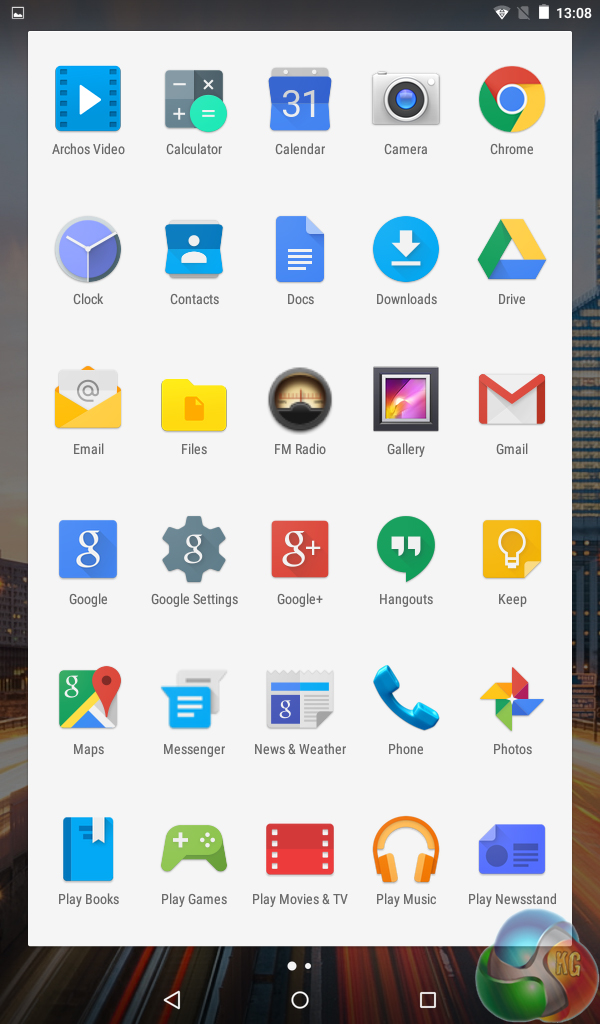This image is a screenshot taken from someone's cell phone. The background of the screen is black, with faint, colorful swirls that are subtly visible. In the lower right corner, there's a semi-transparent, colorful circular blob with the initials "KG" on it.

Dominating the screenshot is a white rectangular grid occupying most of the screen. The grid contains 30 app icons arranged in six rows of five columns each. The apps are organized in alphabetical order. 

Starting from the top row, the first five apps are Archo's Video, Calculator, Calendar, Camera, and Chrome. Moving down, the next row includes Clock, Contacts, Docs, Downloads, and Drive, continuing in a similar structured format down to the last row, where Play Newsstand appears in the lower right corner.